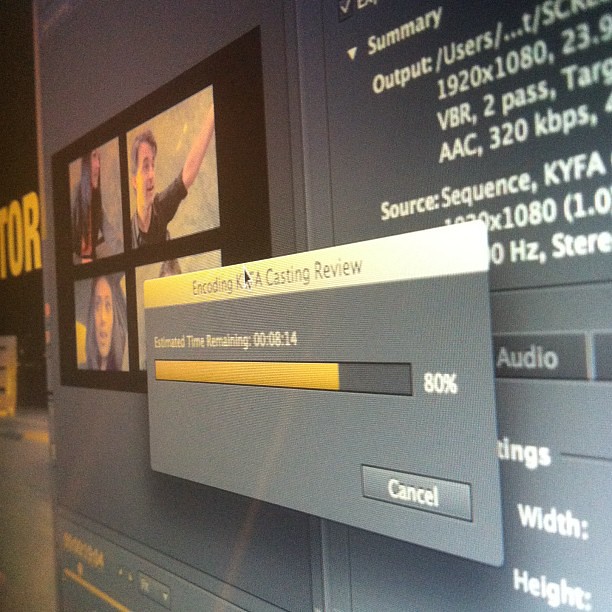The image captures a computer screen, photographed at an angle with the right side of the screen closer to the viewer. The background of the screen is gray, showcasing a video editing application. On the left side, there is a 2x2 grid displaying four faces—two females and two males—presumably part of a casting review. The right side contains detailed information about the images, including options for settings like output, sources, and sequence, as well as dimensions listed as 1920 by 1080.

Superimposed on this background is a dialog box partly obscured by a black mouse cursor, reading "ENCODING K... A CASTING REVIEW." Below this, it estimates the time remaining at 8 minutes and 14 seconds, with a yellow progress bar indicating 80% completion. Additionally, a "Cancel" button is visible beneath the loading bar. The image is slightly blurry, adding to the informal capture style, suggesting it might be taken from a projector or simply a screenshot from another device.